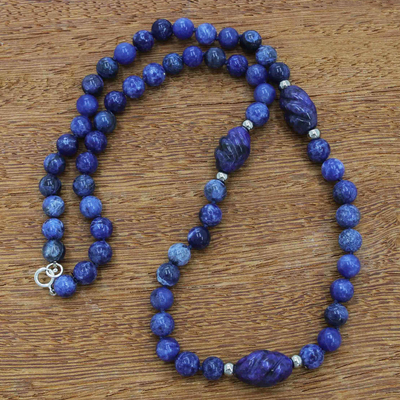The image showcases a short necklace, potentially a choker, elegantly displayed on a medium-grain wooden table. The necklace features a striking design of blue beads, crafted from natural stone, with varying shades from very dark to fairly light blue, giving it a marbled appearance. Three larger decorative blue beads stand out, each framed on either side by two small silver spacer beads, totaling six silver beads adjacent to these prominent stones. The rest of the necklace consists of smaller, round blue beads, creating a harmonious and balanced look. A silver clasp completes the piece, adding a touch of sophistication. For all your beading supply needs, visit Beadaholique.com.